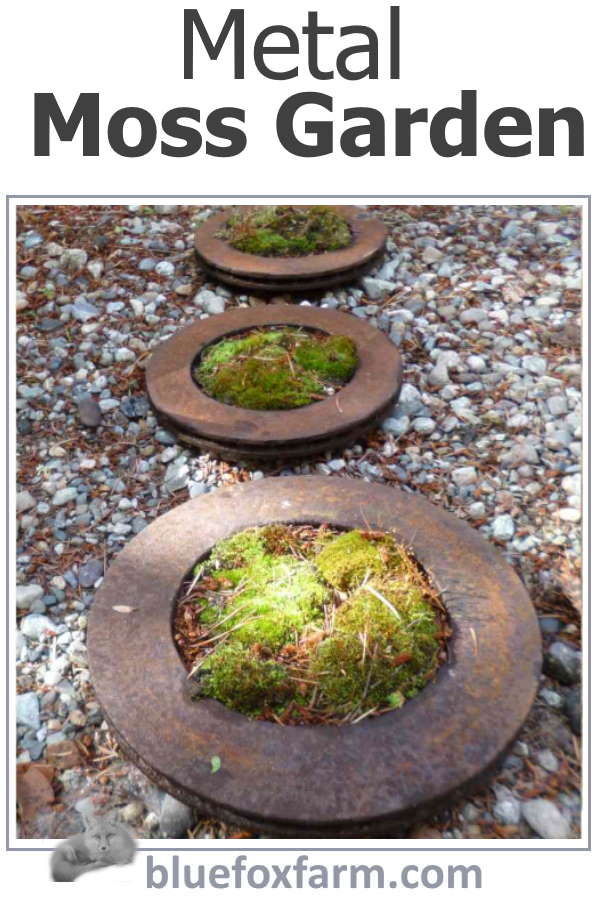This vertical photo captures an outdoor scene featuring three circular metal plant holders. These holders, which have a copper or bronze finish, contain vibrant green moss in their centers. Surrounding the moss is a bed of cedar-colored mulch, enhancing the earthy aesthetic of the arrangement. These objects are positioned amid a ground covered in stones or pebbles, creating a natural backdrop. At the top of the image, the text "Metal Moss Garden" is prominently displayed in black letters. Below the photo, the text "bluefoxfarm.com" is accompanied by a gray fox logo, suggesting that this image is part of an advertisement or promotional material for Blue Fox Farm. The overall color palette includes hues of black, white, gray, brown, light blue, green, and orange.